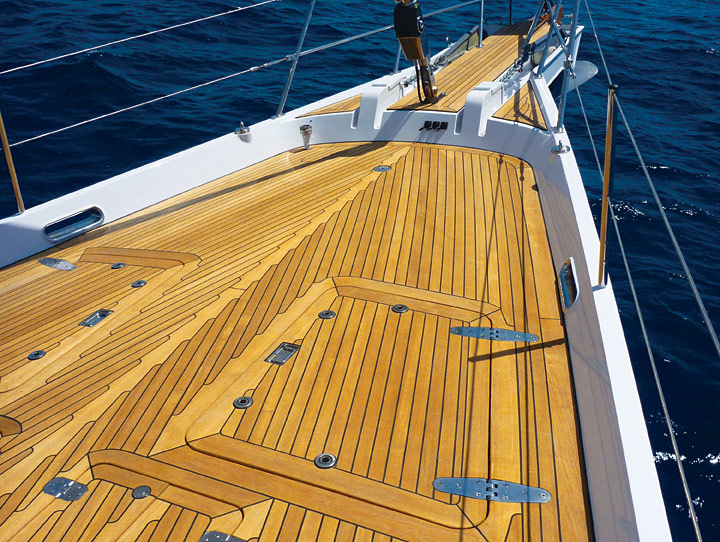The photograph captures the deck of a luxurious, likely new sailboat or yacht, prominently showcasing its meticulously laid wooden floor with a rich, brown hue. The deck's edges are framed by pristine white walls, reflecting the sunlight and giving the boat a highly polished, almost metallic appearance. Adding to the sophisticated design, there are metal joints and wires running along the perimeter of the deck, serving as safety barriers. At the front end of the deck, a long wooden plank extends outward, enhancing the boat’s elegant profile. The vessel is floating on the calm, deep blue waters of what appears to be the ocean, with gentle ripples indicating a slightly choppy yet beautifully sunny day. The sparkling water underscores the serene and picturesque seascape surrounding the yacht.